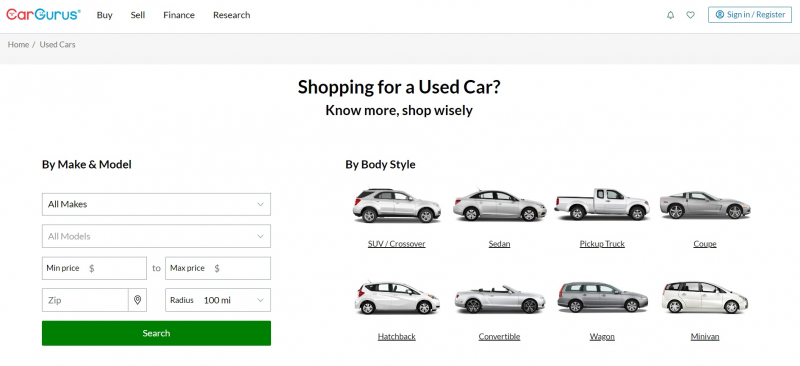A detailed screenshot of the CarGurus website interface is depicted. The CarGurus logo appears prominently in the upper left corner, with "Car" in red and "Gurus" in blue. Next to the logo, on a white background, are navigation options in black text: "Buy," "Sell," "Finance," and "Research." On the far right, the interface includes a blue notification bell icon, a heart icon, and a "Sign In/Register" button outlined in blue. Below the navigation bar, the site offers a selection pathway labeled "Home / Used Cars." The headline in the central area of the page reads, "Shopping for Used Cars? No More, Shop Wisely."

Directly beneath this headline, categorized by body style, are options including SUV, Crossover, Sedan, Pickup Truck, Coupe, Hatchback, Convertible, Wagon, and Minivan, each accompanied by an icon of a vehicle in silver-gray color. On the left side of these categories is a search menu featuring dropdowns for "Make" and "Model," price range selectors labeled "Min Price" and "Max Price," a Zip Code input field with a location marker icon, and "Radius" options currently set to 100 miles. At the bottom of this search menu is a green search button with the word "Search" in white lettering, ready to facilitate the search for used cars based on the specified criteria.